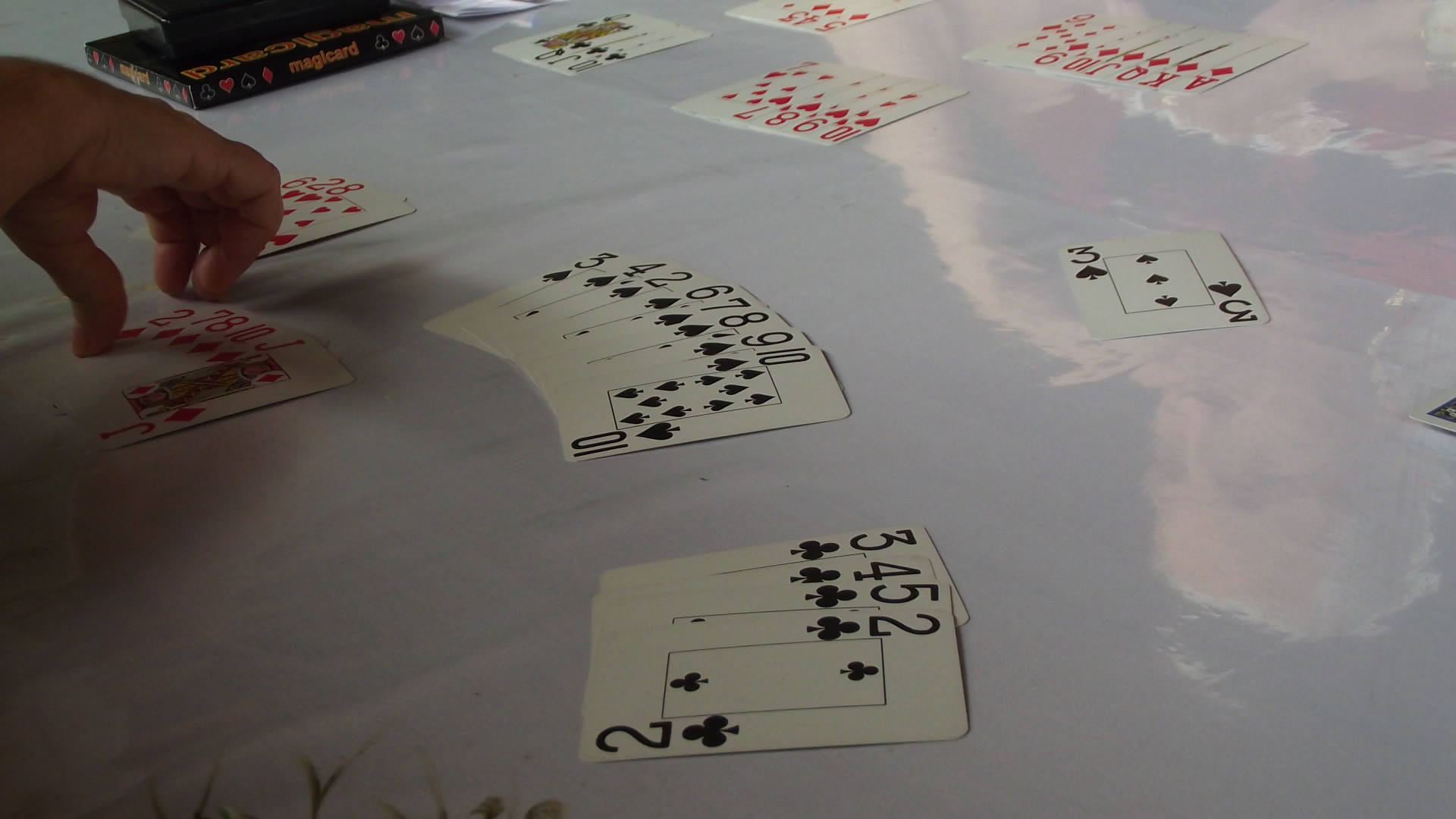This photograph captures a dimly lit scene featuring a highly polished, smooth-surfaced table, possibly used for games or creative activities. The table appears to be a light gray color and is covered with a variety of playing cards. At the top of the image, there is a box labeled "Magic Card," with an additional item stacked on top of it. The left side of the photograph shows a hand reaching for a hand of cards containing the two of diamonds, alongside the seven, eight, ten, and jack of diamonds, all held together.

Throughout the table, various suits are visible. To the middle right of the photo lies a single three of spades. Other spades such as the three, four, two, six, seven, eight, nine, and ten are spread across the table. There is also a sequence of clubs, including the three, four, five, and two. On the top part of the image, facing towards the upper right, there is a series of heart cards—ten, nine, eight, and seven—all arranged in a manner facing another player. Additionally, a complete set of diamond cards, from ace to nine, is scattered across the table.

The overall scene is dark and slightly obscured by the dim lighting, with the glossy surface of the table reflecting the scattered cards and creating a subtle shine.